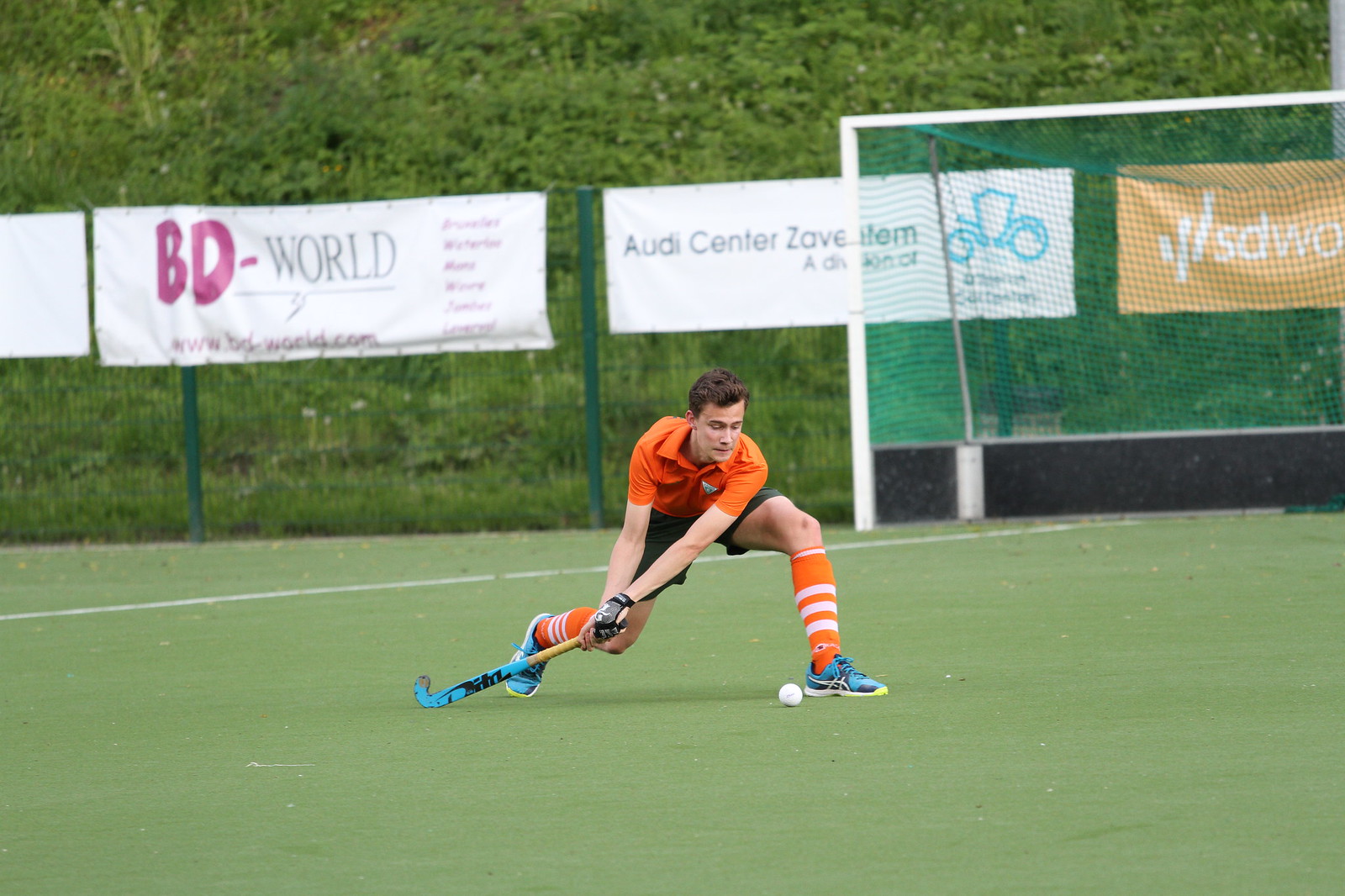The image depicts a male field hockey player poised to hit the ball in front of the goal. He is dressed in an orange uniform shirt, black shorts, and orange knee socks with white stripes. His teal field hockey stick and blue shoes stand out. The player is crouched low, ready to swing, with a gloved hand gripping the stick firmly. Behind the goal, a fence adorned with advertisements can be seen; one sign reads "BB-World," while another, partially obscured, features the words "Audie Center Zave Island" with a small car design. The backdrop includes green grass marked with white chalk lines, a sunny sky, and some hilly trees.